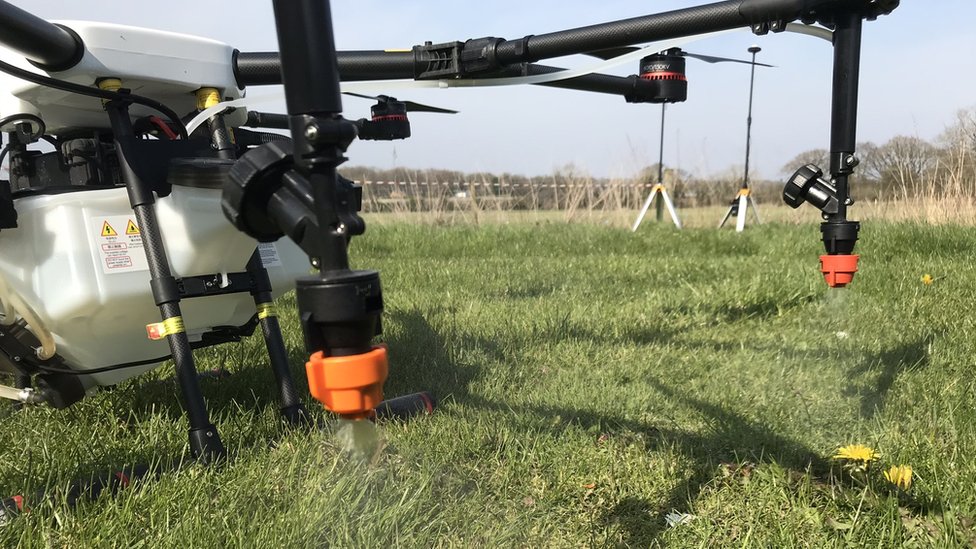This is a close-up, outdoor color photograph of a gas-powered drone situated on a green grassy field, with dandelions scattered around. The drone, which appears to have black metal feet, is resting on the grass. Its body is primarily composed of plastic, with the lower portion made of translucent white plastic containing a visible liquid. The drone features a black motor mounted on the top. Extending outward from the body are black pipes that support rotor blades, which are white in color. Visible at the forefront of the image are some of these blades. The background reveals a blue sky with a tree line and houses just beneath the horizon. The object, evocative of aeronautical machinery, has small propellers, and possibly a fuel tank that features some orange detailing, enhancing its mechanical appearance.